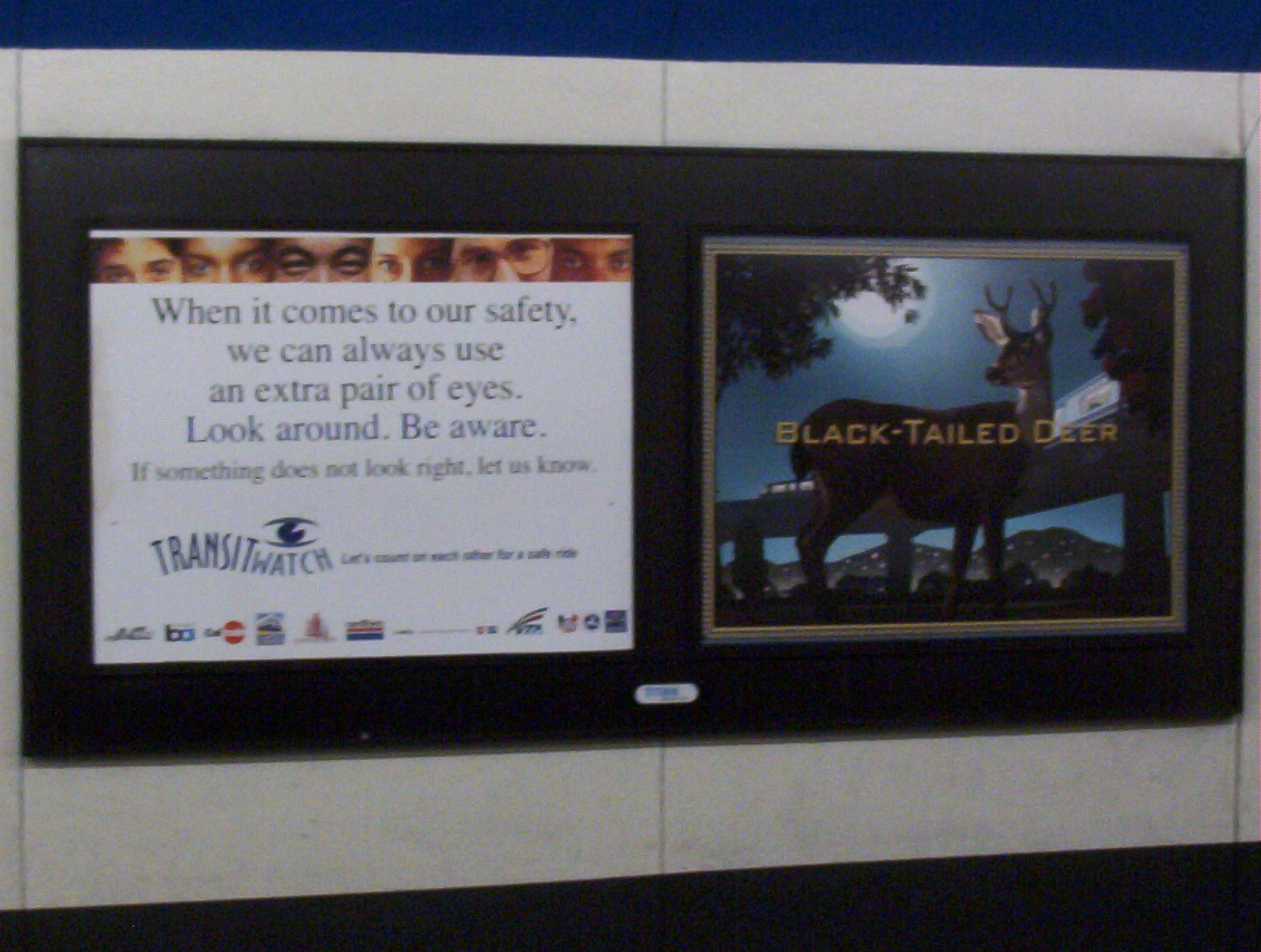The image depicts two side-by-side advertisements on the wall of a subway station. The advertisement on the left has a white background and features a row of six photographs at the top, displaying only the eyes and foreheads of ethnically diverse individuals, some wearing glasses. Below the photos, the text reads, "When it comes to our safety, we can always use an extra pair of eyes. Look around, be aware. If something doesn’t look right, let us know. Transit Watch. Let's count on each other for a safe ride." Beneath this message, there are several logos, likely representing company sponsors including the BART system.

The advertisement on the right presents a painting of a black-tailed deer standing in front of a bridge under a moonlit night. Over the image, yellow text states, "Black-Tailed Deer."